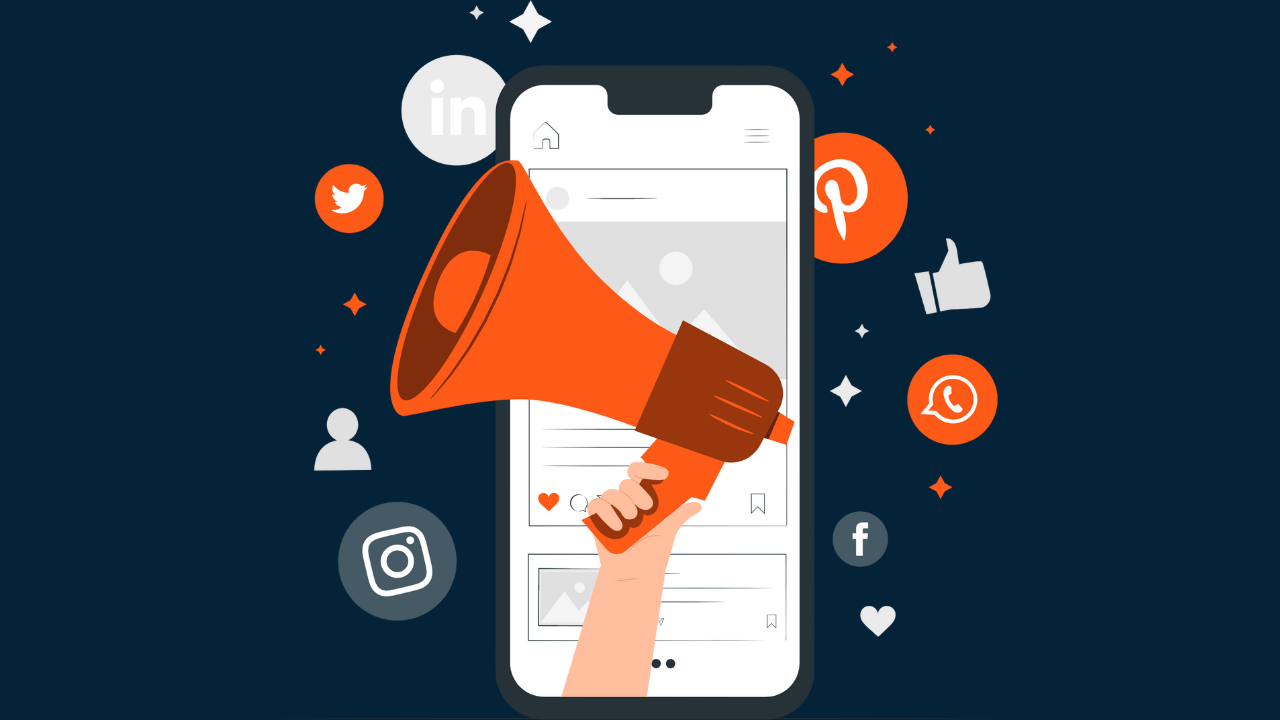The image is a graphic design with a navy blue background, featuring a centrally located rendering of a smartphone displaying a screenshot reminiscent of a social media app, identifiable by the presence of a red "like" button and black lines against a white screen. Surrounding the smartphone are various monochromatic social media logos within colored circles: Twitter and WhatsApp logos in orange circles, Facebook and Instagram logos in gray circles, and LinkedIn's logo in a light gray circle. Additional decorative elements like differently sized stars dot the background. Emerging from the lower portion of the image, a drawn arm holds an orange megaphone pointed toward the upper left corner, symbolizing the amplification of voices through these social media platforms.